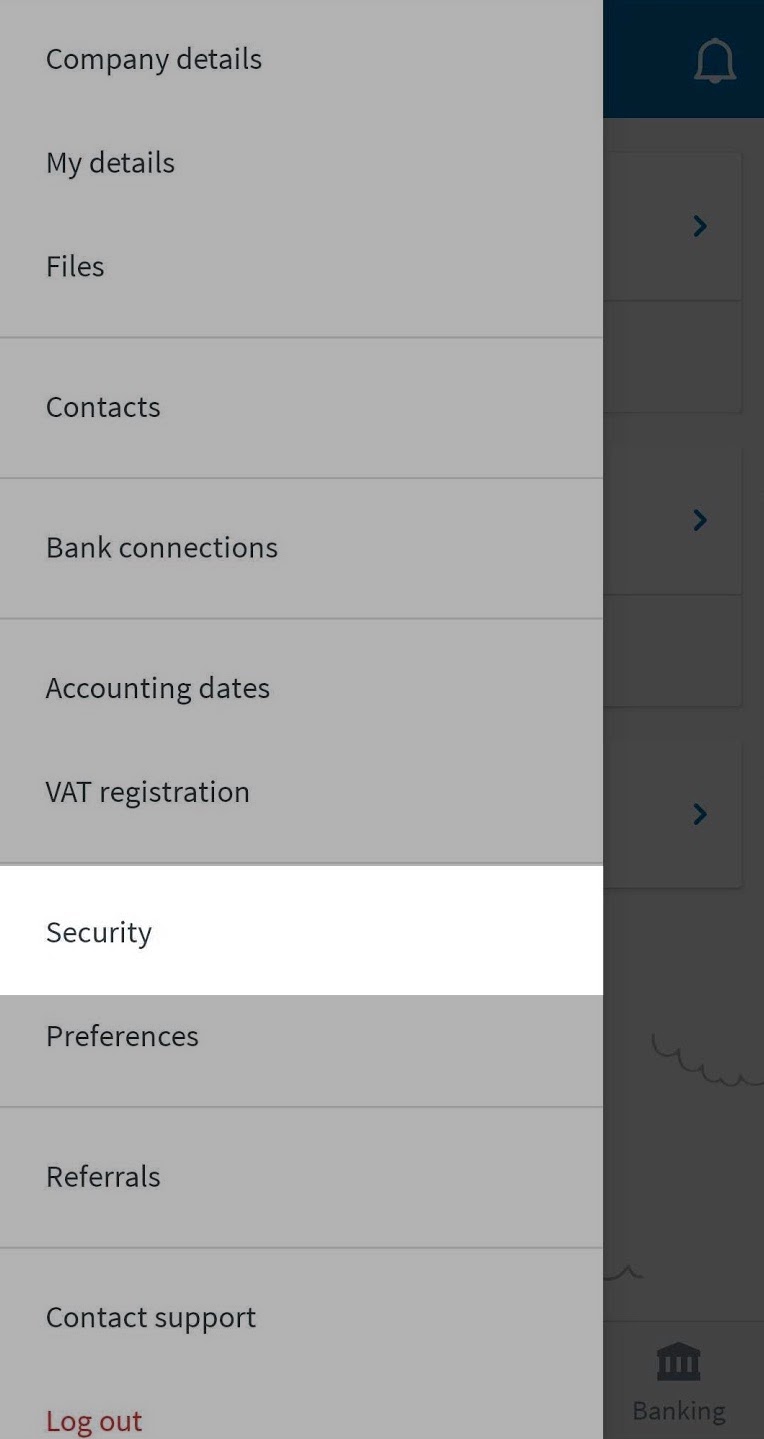The image depicts a mobile phone screen displaying a pop-up menu from a web application. The interface offers a range of options including "Company Details," "My Details," "Files," "Contacts," "Bank Connections," "Accounting Dates," "VAT Registration," "Security," "Preferences," "Referrals," and "Contact Support." At the bottom of the menu, there is a red "Log Out" button. The "Security" option is highlighted in white, indicating it has been selected.

Only a small portion of the underlying page is visible, suggesting that another section is partially obscured by the menu. The screen shows a notification area with no active alerts, highlighted by three left-facing arrows. Additionally, there's a section labeled "Banking," accompanied by a bank icon at the bottom of the screen. Above this area, the background features a series of squiggly lines resembling hand-drawn clouds. 

The overall design utilizes a predominantly gray and dark gray-black color scheme, maintaining a neutral aesthetic with the exception of white highlights to indicate the selected menu option.